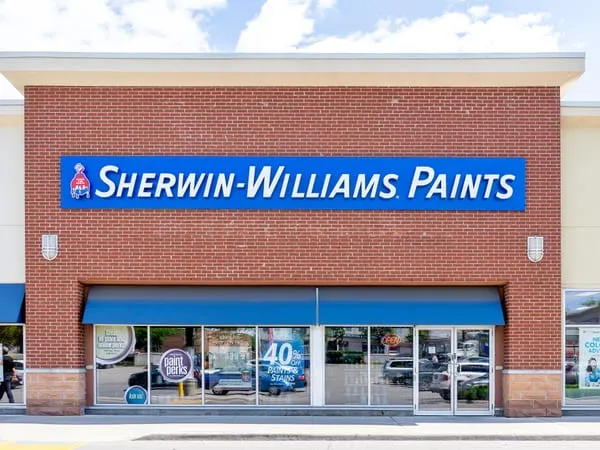The image showcases the front facade of a red brick building with distinct architectural features. The building has a prominent white roof, complemented by white pillar-like structures on both the left and right sides. A row of glass windows spans the front of the building, beneath an inviting blue canopy overhang. Centrally positioned on the front brick wall is a blue sign that proudly displays "Sherwin-Williams Paints" in bold white letters. To the left of the text, the iconic Sherwin-Williams logo features a globe being enveloped by a can of red paint. Flanking the sign are two gray lights, symmetrically placed, one on each side. On the glass window, a prominent emblem advertises a "40% off" promotion. In the reflection of the window, the parking lot can be faintly seen, adding depth to the image.